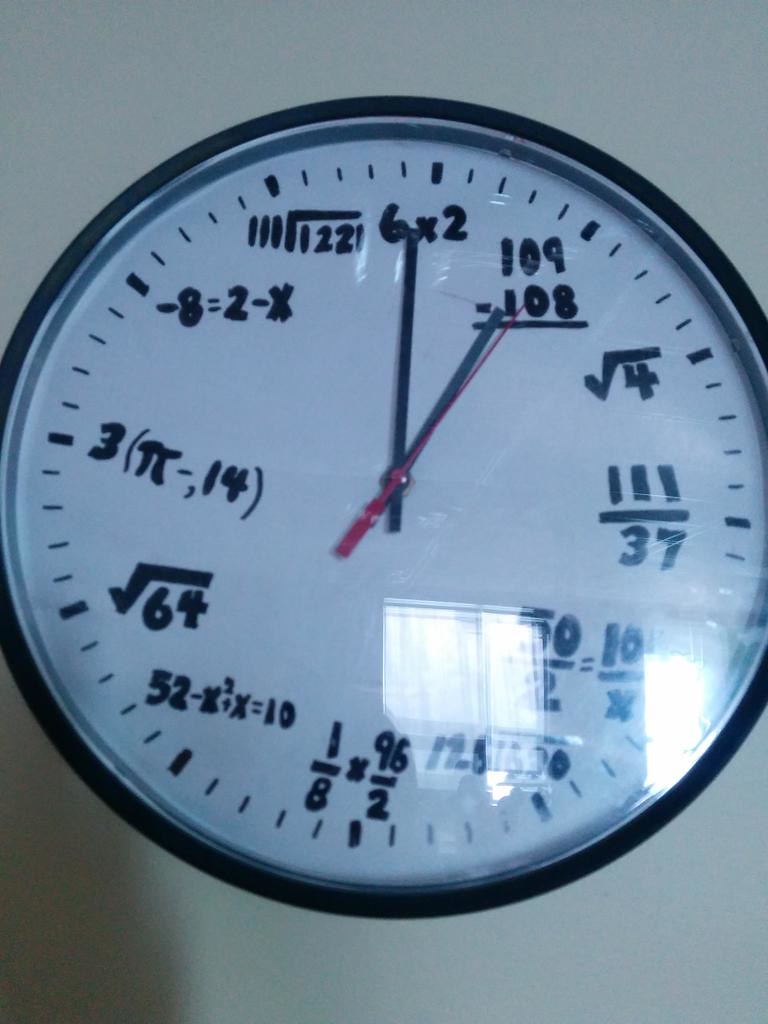The image features an intricate close-up of a unique wall clock, set against a stark white wall. The clock's border is a solid black rim encircling its minimalist design. The face of the clock is a clean, sharp white adorned with fine lines marking each hour, with every bolded line corresponding to an hour of the day. Remarkably, instead of traditional numbers, each hour is represented by a mathematical equation. For instance, the position for 12 o'clock shows "6 x 2," while 1 o'clock is illustrated by "109 - 108." The 3 o'clock mark features the square root of 4 (√4), and 4 o'clock is depicted with "37 ÷ 111." However, a bright glare from a window obscures the section where the 4 and 5 o'clock markings would be, making those equations indecipherable. The equation for 6 o'clock reads "(1 ÷ 8) x (96 ÷ 2)." Each position around the clock face similarly features a diverse array of mathematical expressions, inviting viewers to solve them in real-time. The overall aesthetic of the clock blends the simplicity of its color scheme with the intellectual challenge posed by its unique numeric representations.